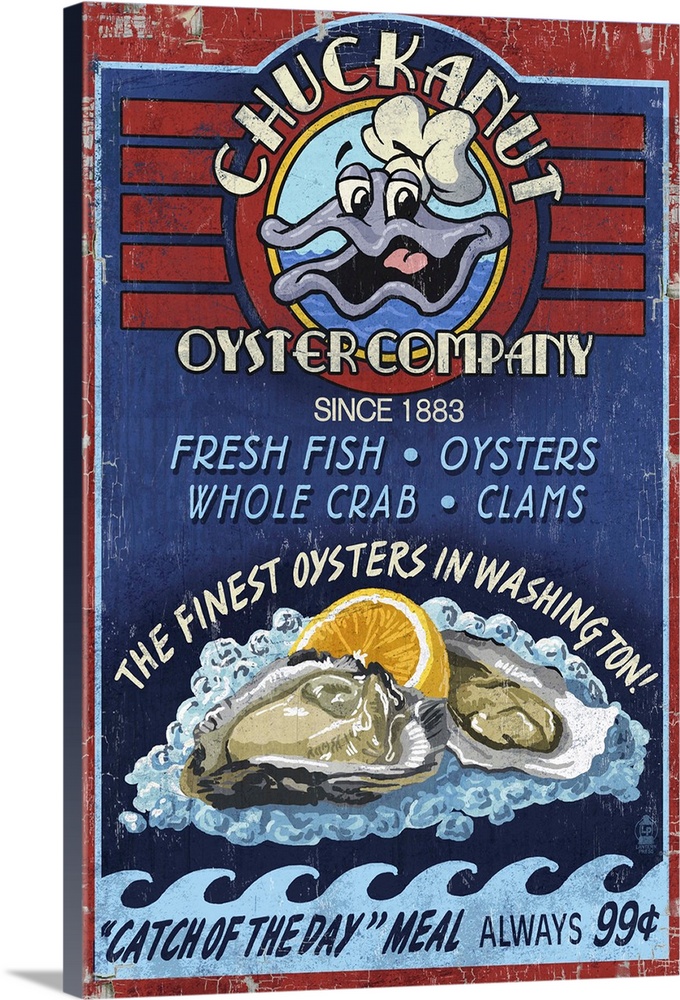The image depicts a tall, portrait-layout wooden sign advertising the "Chuck-A-Nut Oyster Company" established in 1883. The sign boasts a predominantly blue background with a red border on top. The top section features the company’s logo: a round circle with a smiling clam donning a white chef's hat, a light blue sky-like background at the top, and a darker blue wave pattern below. Above the logo, large white text proclaims "Chuck-A-Nut." Below the logo, white text states, "Oyster Company Since 1883," followed by blue text listing "Fresh Fish, Oysters, Whole Crab, Clams." Further down, it proudly declares in white, "The Finest Oysters in Washington." An illustration beneath this text shows two halved oysters and a lemon wedge resting on ice. At the bottom of the sign, dark blue text over a light blue wave-patterned background advertises the "Catch of the Day Meal, Always 99 Cents."